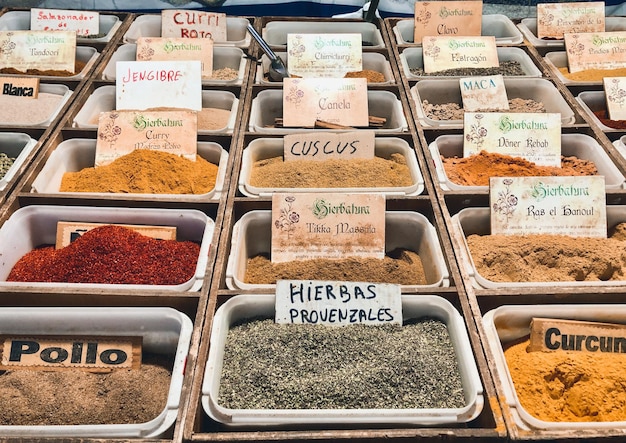The image is a close-up photograph of a display table at a spice store, showcasing several bins of herbs and seasonings. The bins are arranged in neat rows within brown wooden frames, creating a visually appealing and organized arrangement. Each bin is a rectangular white plastic container with slightly rounded corners and a snap lid design. Nestled inside the bins are various vibrant powders and granules, each distinctly colored in shades of gray, yellow, brown, red, orange, and beige.

Labels with the names of the spices are clearly visible, though some appear handwritten and harder to read. Among the legible labels are Curry, Curry Roto, Jenbury, Palo, Blanca, Herbas Provenzales, Couscous, Canela, Cherrisburg, Clove, Maka, Donner Rebob, Ross L., Hanul, and Curcumin. The overall setting of the photograph radiates the charm and diversity of a seasoning store, highlighting the rich variety and vivid colors of the spices on display.